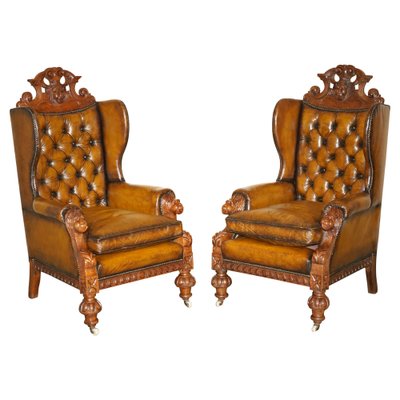The image features two identical Victorian-style armchairs made of brown leather and detailed wood, positioned diagonally toward each other on a stark white background. The chairs exhibit a rich caramel brown hue, with the leather appearing to be in excellent, almost pristine condition. Each chair features a high back with tufted leather, crowned by an intricately engraved wooden piece reminiscent of a regal design. The armrests are complemented by curved wooden supports and adorned with engraved wood accents at the ends. The front legs are elegantly spindled, while the back legs are straight, providing a subtle contrast in their craftsmanship. The leather cushions add an extra layer of comfort to the seats. The overall elegance and detailed workmanship suggest a setting suitable for a formal library or similar refined environment.